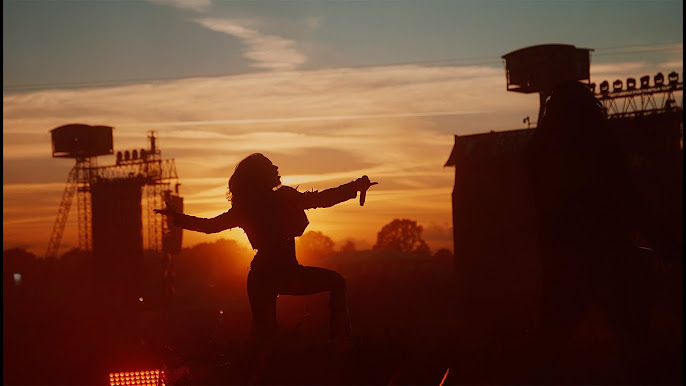The image captures an outdoor scene at sunset, characterized by a sky with a gradient of light blue at the top, transitioning to orange and yellow hues near the horizon due to the setting sun. The sky features elongated tendrils of clouds stretching upward and a sweeping formation moving from right to left, illuminated with the warm colors of the fading sunlight.

In the foreground, a woman is gracefully dancing, her silhouette stark against the radiant backdrop. She strikes a dynamic pose with one knee bent, the other leg straight, and both arms extended as if holding imaginary objects. Her long hair flows down her back, and she gazes upwards with her face turned slightly to the right, creating an air of joyous performance or playful spontaneity.

On the left side of the image, there is a large cylindrical tower structure with metal beams supporting a boxy shed or building at the top. The right side features a similar industrial-style building with a squared tower atop a framework of beams. The background horizon is lined with trees, and the overall scene suggests an industrial area, perhaps reminiscent of a festival setting in the desert, with the arising silhouette effect due to the contrast of the dimming light against the structures.